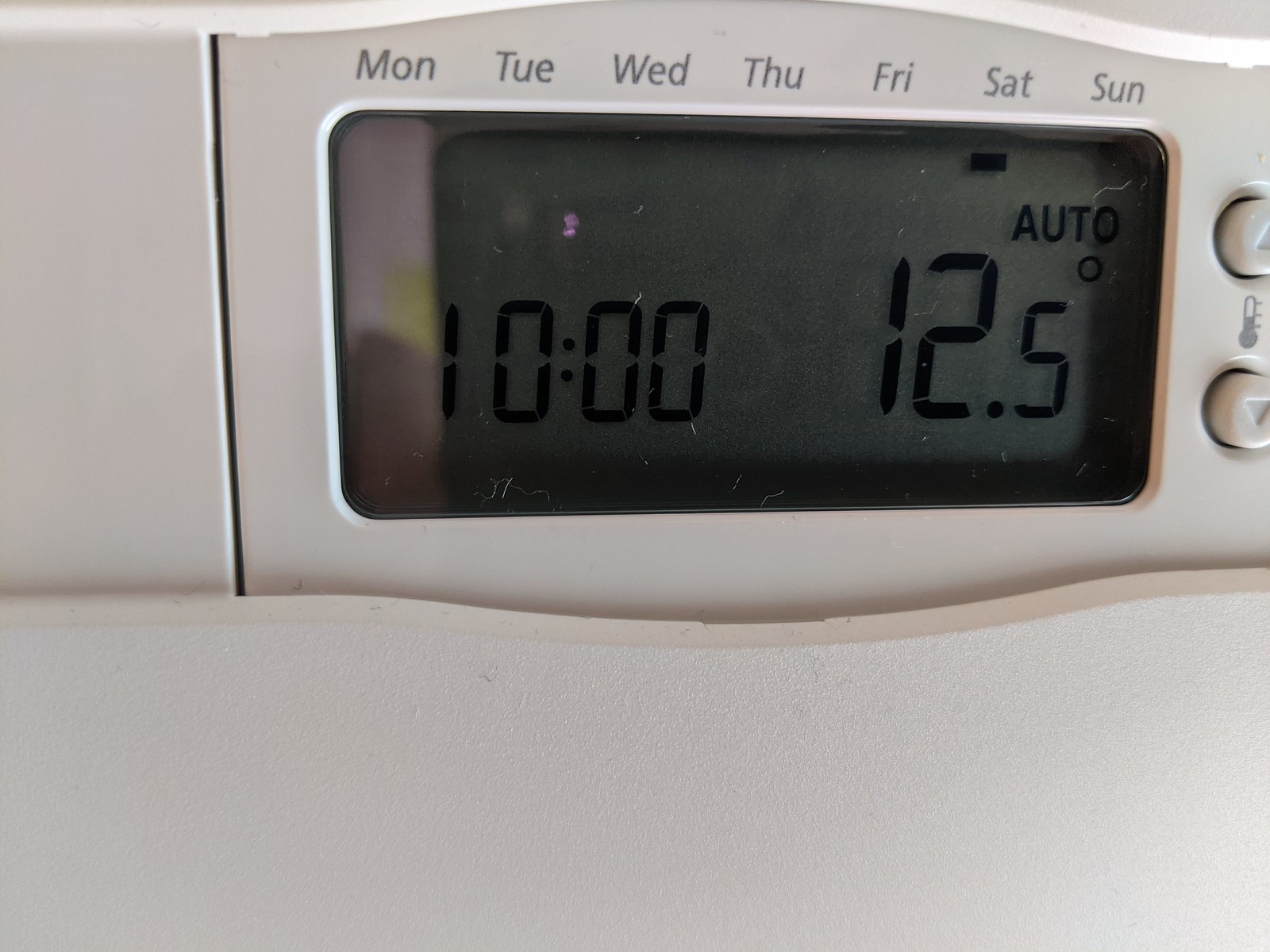This detailed close-up photograph captures an intricate view of a white digital thermostat or climate control device, occupying the entirety of the image. The focus is primarily on the upper section, where a rectangular, gray digital display is encased in a glass protector. 

The display showcases the days of the week across the top, listed as Monday through Sunday. The current time is prominently displayed as 10:00, without indicating whether it is a.m. or p.m. Adjacent to the time display, there is a small solid black rectangle, possibly indicating battery status. Below this, the display reads "Auto" alongside a degree symbol next to the numbers 12.5, likely representing the current temperature setting.

To the right of the display are two circular white buttons, each adorned with a triangular symbol. The upper button's triangle points upward, suggesting it increases the temperature or settings, while the lower button's triangle points downward, indicating it reduces them. Between these two buttons is a partially grayed-out thermometer icon, symbolizing adjustments in temperature or airflow.

A subtle reflection in the display hints at an indistinct yellow object in the background, adding a slight shadow or hue to the otherwise monochromatic panel.